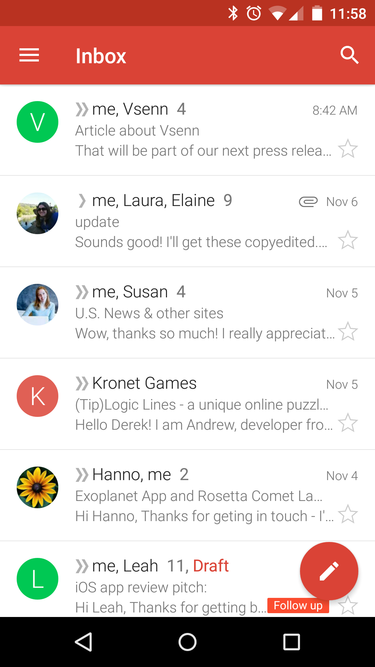This image depicts a mobile interface of a person's email inbox with various UI elements and notifications. At the very top, the notification bar indicates active Bluetooth, an alarm set, phone reception, battery level, and the current time. This section is highlighted in a darker red, while a lighter red bar underneath features three horizontal lines representing a hamburger menu on the left, the word "Inbox" in the center, and a magnifying glass icon for search functionality on the right.

The main background beneath these bars is white, showcasing a list of six email conversations. Each email thread displays specific details:

1. The first conversation has a total of four emails.
2. The second conversation is more extensive, containing nine emails.
3. The third conversation also includes four emails.
4. The fourth is a singular, standalone email.
5. The fifth conversation consists of two emails.
6. The sixth and final email thread is marked as a draft and is labeled for follow-up.

This detailed view offers a comprehensive look at the person's current email interactions and organizational labels for efficient email management.